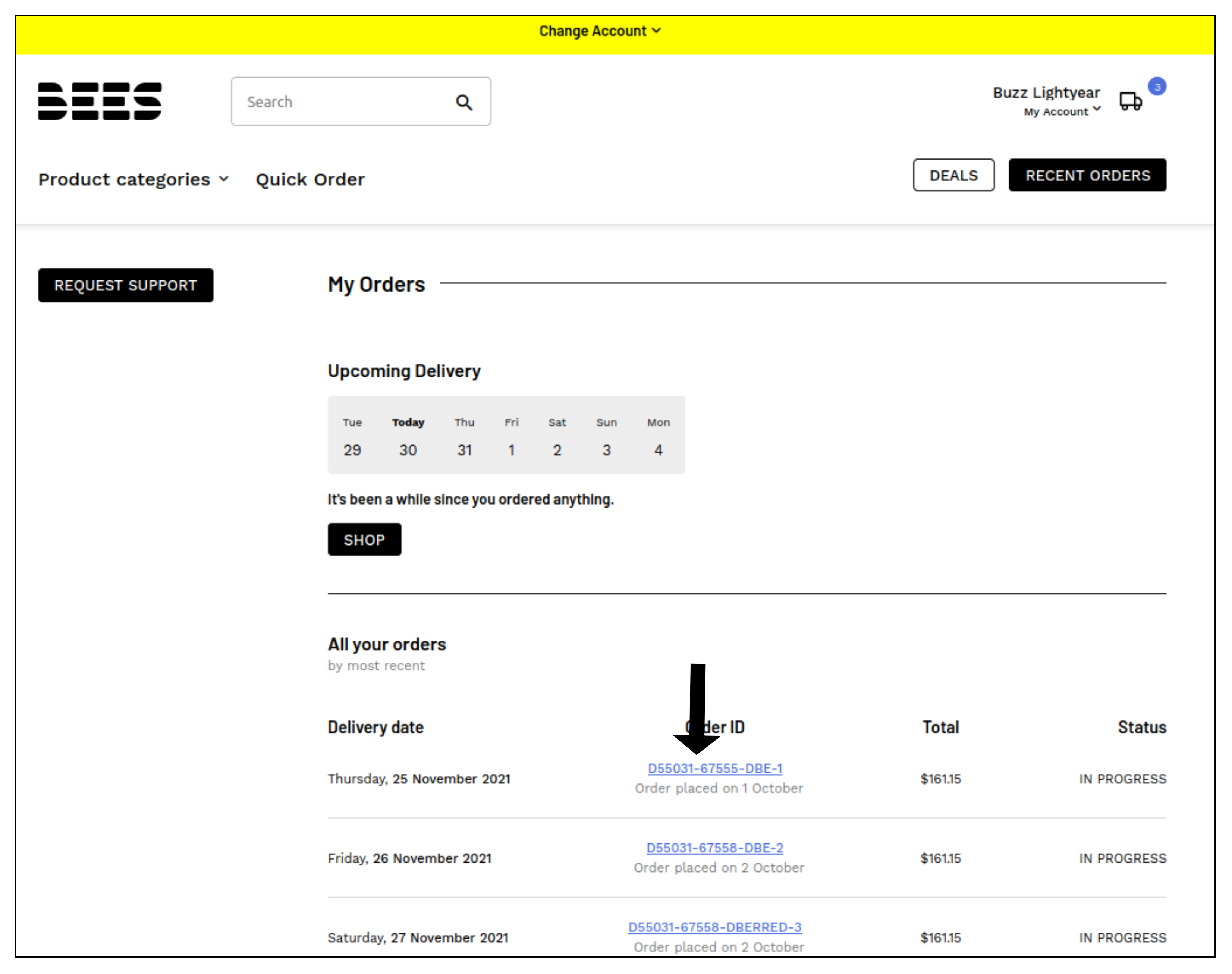The image displays a detailed and organized online order management interface. 

At the top, a prominent yellow bar displays the notification "Change account" with a search bar beside it, identified by a magnifying glass icon. Adjacent to the search bar, the words "Product Categories" and "Quick Order" can be seen.

On the top right of the interface, there are various labeled icons. "Buzz Lightyear" is the first, followed by "My Account" marked by a truck icon. A small white circle with the number three in it indicates multiple notifications or messages. Next to it, a white box labeled "Deals and Recent Orders" is visible. A blue and black rectangle button labeled "Request Support" is prominently placed nearby.

The section titled "My Orders" highlights upcoming deliveries. A gray rectangular box details the delivery schedule, listing Tuesday, Thursday, Friday, Saturday, Sunday, and Monday as delivery dates.

A text prompt indicates, "It's been a while since you ordered anything. Shop all your orders by most recent delivery date."

Below this, specific order details are listed as follows:

- Order ID D55031-6755-DB1, placed on October 1st, with a total amount of $161.15, marked as 'In Progress.' The expected delivery date is noted as Friday, November 26, 2021.
- Another order, ID D55031-67558-DB21, also for $161.15, is listed with a delivery date of Saturday, November 27, 2021.
- A third order, ID D45021-6758-DBED3S3, placed on October 2nd for $161.15, is similarly marked 'In Progress.'

The interface also includes directional cues, such as a black arrow pointing towards blue text, which appears to be a hyperlink or actionable item.

Overall, the interface efficiently provides a comprehensive overview of order statuses, upcoming deliveries, and account management features.